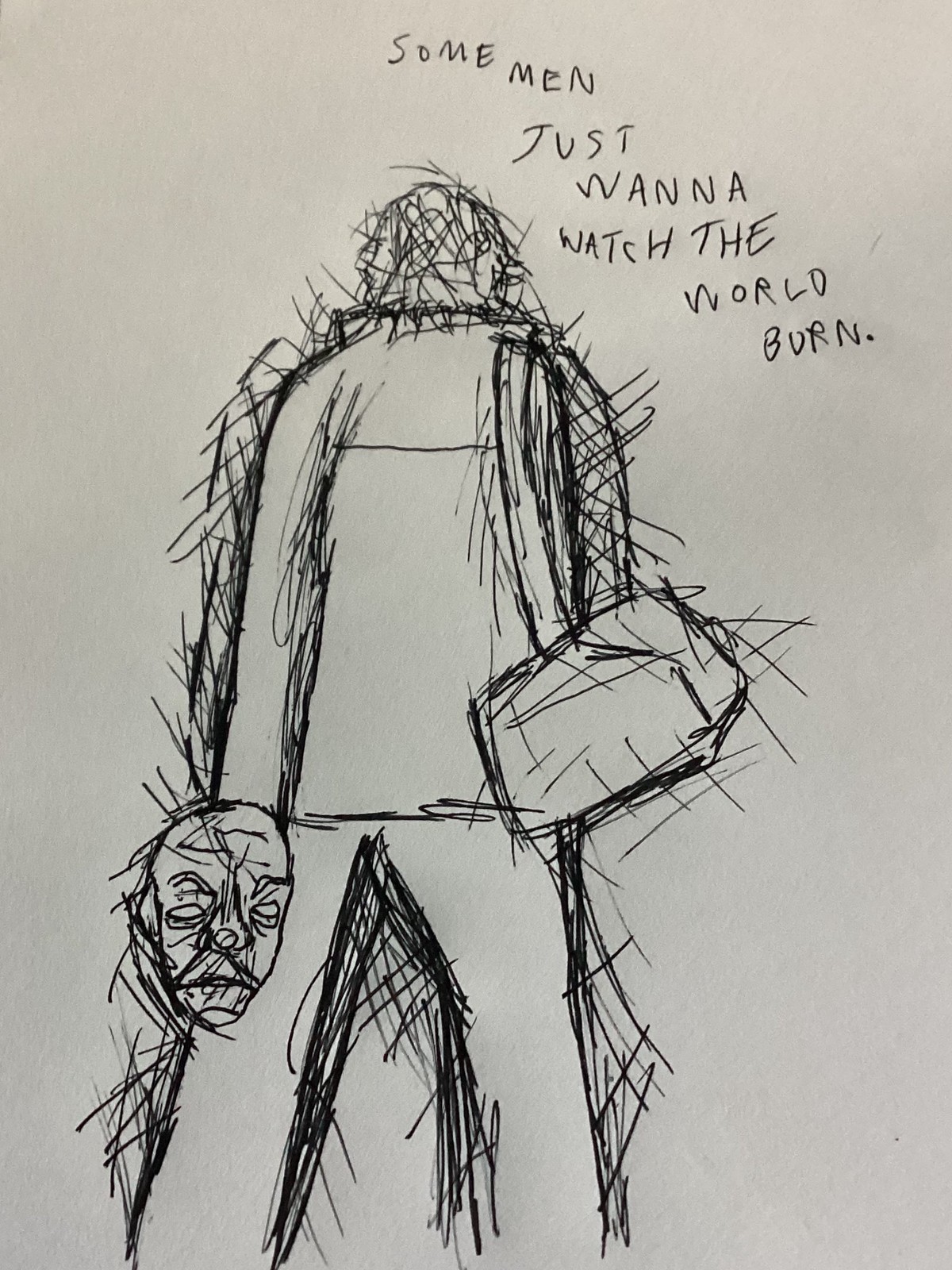A rough sketch on light gray or beige paper depicts a faceless man drawn with chaotic black ink lines, creating a scratchy and abstract appearance. The man, viewed from the back, wears a long-sleeved jacket and pants. In his left hand, he holds a mask with exaggerated features, including empty eye sockets, pronounced eyebrows, and a frowning mouth. His right hand appears to carry a bag or satchel with a strap over his shoulder. Above the sketch, in capital black ink letters, the text "SOME MEN JUST WANT TO WATCH THE WORLD BURN" extends from the upper left to the lower right of the paper, adding a sinister context to the imagery.